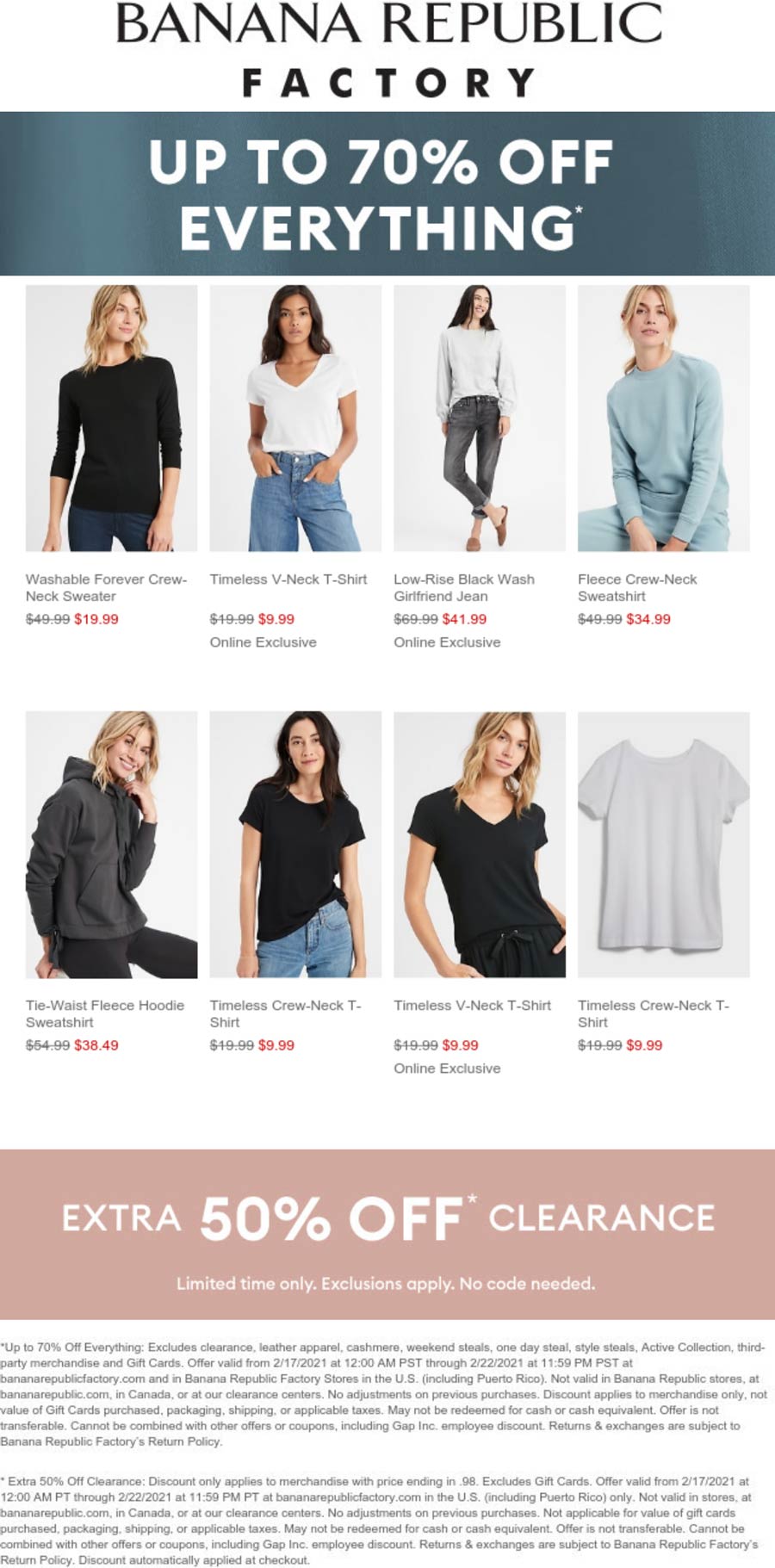The image appears to be a promotional advertisement for Banana Republic. At the top, in bold capital letters, is the brand name "BANANA REPUBLIC," followed by the word "Factory" in smaller, yet still capitalized, black text in a different font style. Just below, there's a striking blue rectangle with bold, white capital letters announcing "UP TO 70% OFF EVERYTHING."

Beneath this banner, there is a grid of eight distinct images showcasing various individuals modeling Banana Republic attire. In the top row, from left to right, the first image features a blonde woman dressed in a long sleeve t-shirt and jeans. Next is a woman with a beige complexion and long black hair sporting a short sleeve t-shirt and jeans. Following her is another woman with long black hair and a fair complexion, wearing a white blouse and jeans. The last image on the top row shows a blonde woman in a long sleeve t-shirt paired with blue sweatpants.

In the second row of images, starting from the left, there is a blonde woman wearing a black hoodie and black pants. She is followed by a woman with black hair, wearing a short sleeve black t-shirt and jeans. Next to her is a blonde woman in a short sleeve black t-shirt. The final image on this row is a white t-shirt displayed against a plain white background.

Beneath these images, a pink box highlights an "EXTRA 50% OFF CLEARANCE" offer. At the very bottom of the advertisement, there is a block of small black text, likely detailing terms and conditions or additional information about the sale.